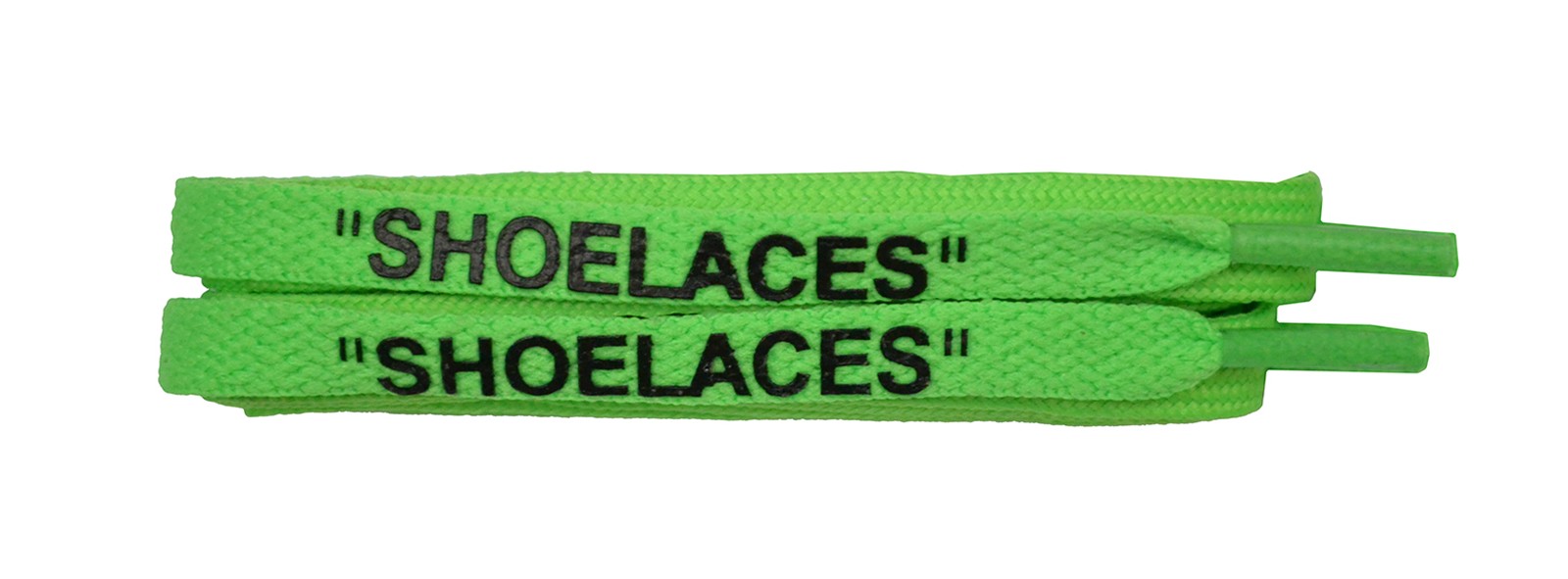This image displays a set of neon green shoelaces folded in a Z-pattern and laid horizontally, one on top of the other, against a clean white background. Each shoelace prominently features the word "SHOELACES" in bold black uppercase letters enclosed in quotation marks, a distinctive design element associated with the fashion brand Off-White. Both shoelaces have slightly darker neon green aglets at their ends to prevent fraying and ease threading. The simplistic composition highlights the vibrant color and branding of the shoelaces, suggesting they may serve as replacements for Off-White designer shoes or merely as a showcase of the brand's unique design.